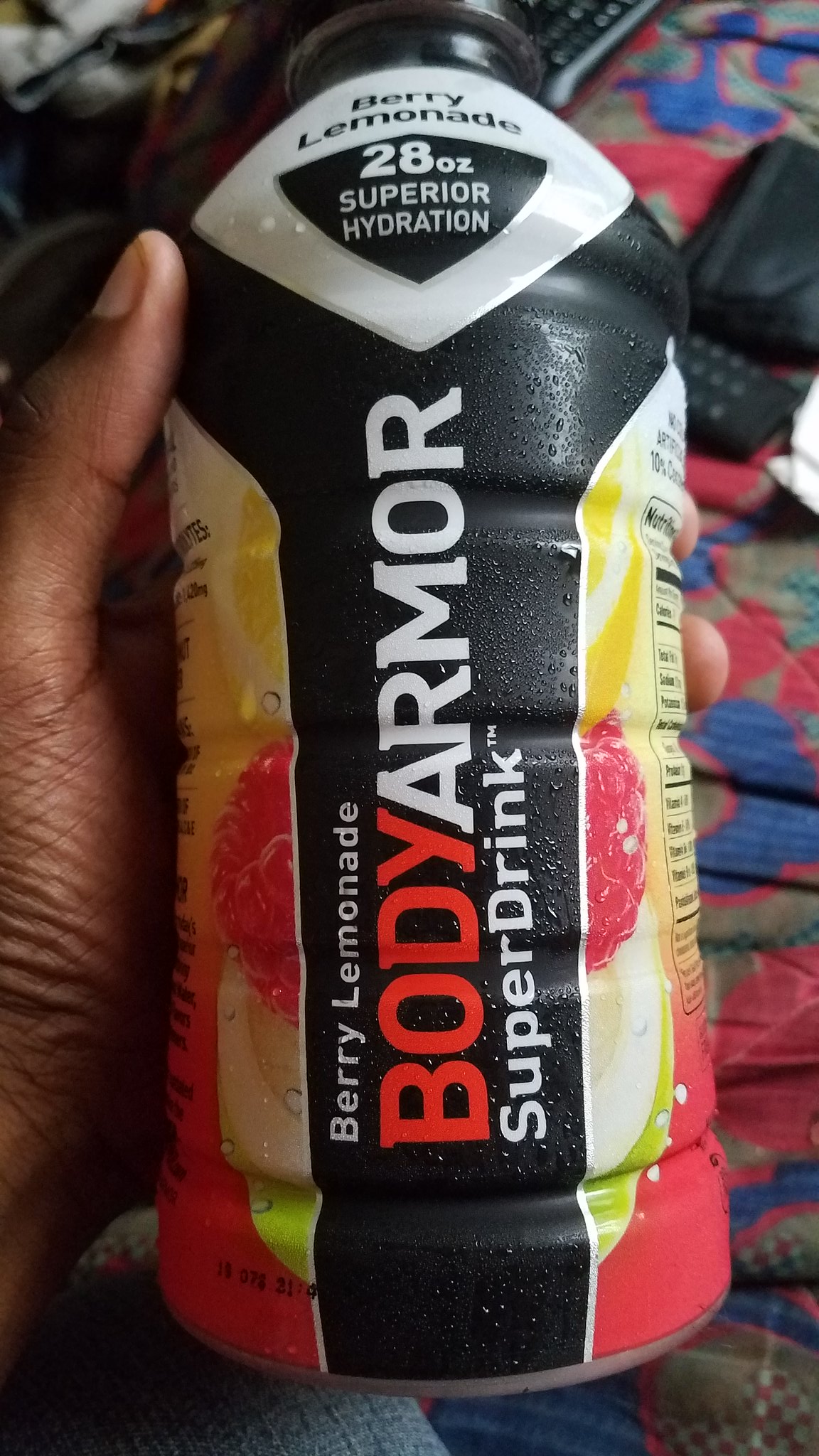A detailed photograph captures the left hand of a black person, displaying the wrinkles indicative of an older male, firmly grasping a large, 28-ounce bottle of Berry Lemonade Body Armor Super Drink. The bottle, made from thick plastic, is further encased in a vibrant wrap. This wrap features a bold black stripe running vertically down the center, flanked by bright, fruity berry colors on either side. The label prominently showcases "Body Armor Super Drink" in white text, with "Berry Lemonade" also labeled in white and parts in red. At the very top, a white section with a black triangle boasts the promise of "28 ounces Superior Hydration." The bottle is topped with a black twist-off cap. In the background, the setting reveals a multicolored bedspread with red, blue, gray, brown, and green hues. Surrounding elements include what seem to be a colorful duvet pile, a black bag, a white piece of paper, some blue jeans positioned in the bottom left, and a remote control visible in the top right.